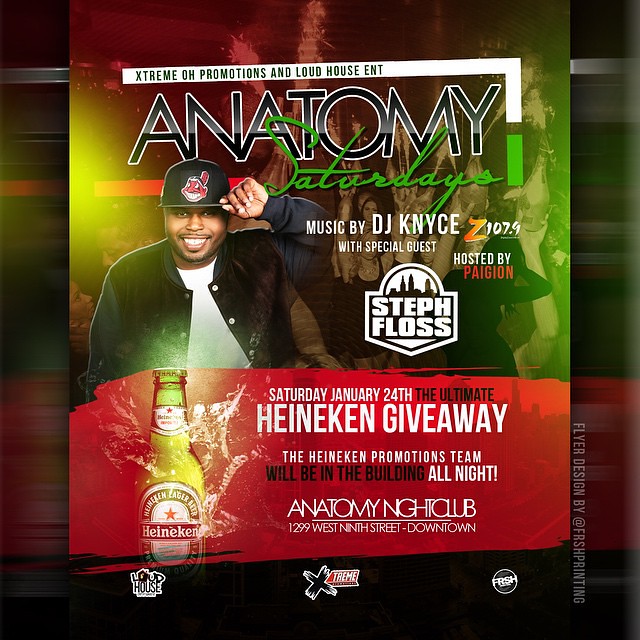This is a detailed flyer advertising "Anatomy Saturdays," a special event at Anatomy Nightclub located at 1299 West 9th Street, downtown Cleveland, Ohio. The top section prominently displays “Anatomy” in large, all-caps black font with a white outline, and “Saturdays” in a bright green, stylized cursive font. The background of the flyer appears wooden.

On the left side of the flyer, there's a smiling African American man wearing a Cleveland Indians baseball cap, a black jacket, and a white t-shirt. He has a thin mustache and some scruff on his chin, with his left arm bent and hand touching the brim of his hat. To the right of his image, it mentions music by DJ Knyce (K-N-Y-C-E) and displays the Z107.9 logo along with another logo for special guest Steph Floss, featuring a cityscape background.

The lower portion of the flyer, set against a red background, promotes the "Ultimate Heineken Giveaway" on Saturday, January 24th. This section highlights a Heineken bottle with water splashing around it on the lower left side. The text indicates that the Heineken promotions team will be present all night. It also lists the event’s address and mentions that the event is hosted by Paigion (PAIGION).

At the very bottom, there are three smaller logos, including Loud House Entertainment and Extreme Entertainment. In the lower right corner, there's a note in a lighter, smaller font, oriented at a 90-degree angle, crediting the flyer design to @FRSHprinting.